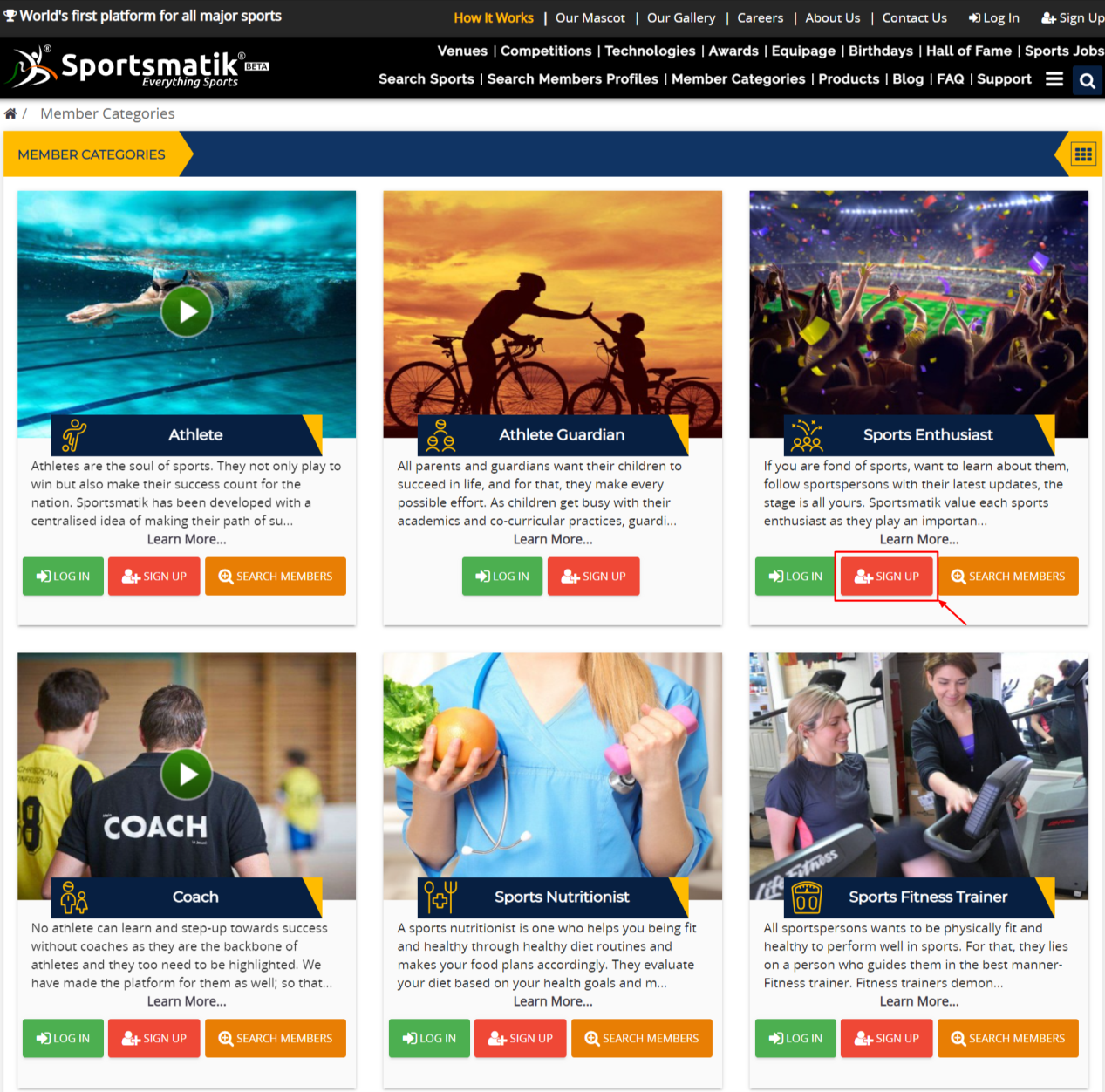A comprehensive and detailed shot against a clean, white background showcasing SportsMatic—the world's first all-encompassing platform for major sports. The interface features an engaging blue header with various sections such as "About Us", "How It Works", "Our Mascot", "Our Gallery", "Careers", and "Contact Us". Navigation is facilitated through options for "Login" and "Sign Up".

The platform is packed with functionalities including venues, competitions, technologies, awards, and equipage information. Users can explore special segments like birthdays, the Hall of Fame, sports job opportunities, and search features for sports and members. There are detailed member profiles and categorized member information.

Upon scanning the interface, users will notice an intuitive layout, highlighted by blue squares arranged in three rows of three, organizing the member categories. The first section prominently displays a video symbol, inviting users to play a video under the category "Athlete". The second section shows a child and an adult riding a bike, categorized under "Athlete, Guardian". All elements aim to provide a seamless and informative user experience, enhanced by icons like the hamburger menu and magnifying glass for easy navigation and search functionality.